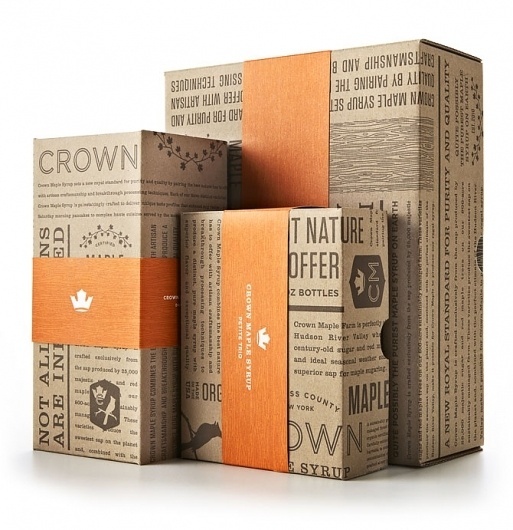The photograph features three rectangular cardboard boxes of varying sizes, all branded with the same design and text: "Crown Maple Syrup Petite Trio." The boxes are displayed on a flat, empty surface with a solid white background, creating the effect of them existing in a white void. This style of presentation is typical for commercial photography, such as for online listings or e-commerce websites. The leftmost box has multiple lines of text printed on it, with "Crown" at the top. Each box features an orange band encircling the middle, adorned with a white crown logo. The white background fills most of the image, making the boxes the central focus.